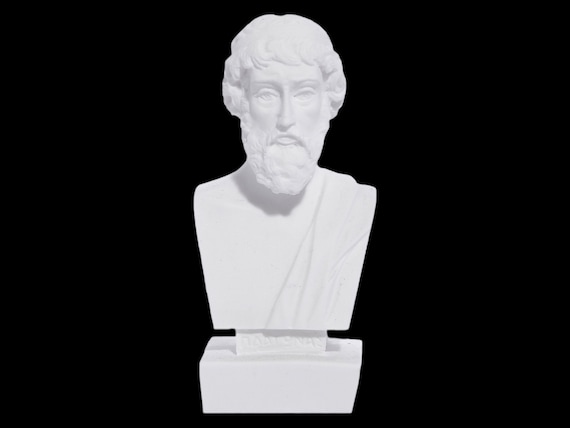The image features a white porcelain-like bust of a man set against a solid black background. The sculpture, positioned centrally, is mounted on a square white base and depicts the torso and head without arms. The man's face is front-facing, characterized by wide eyes, a slightly open mouth, a long beard that reaches the bottom of his neck, and short wavy hair that falls to his ears. He has a thin mustache that sits above notably full lips. There are sculpted details of a toga draped over one shoulder, and subtle wrinkles are carved into the material. The overall appearance of the bust bears a resemblance to Dick Van Dyke, especially in terms of hairstyle and facial features. Below the torso, there is some illegible lettering etched into the base. The smooth surface and clean details suggest a craftsmanship that does not appear carved, enhancing the ethereal, almost pristine quality of the statue.